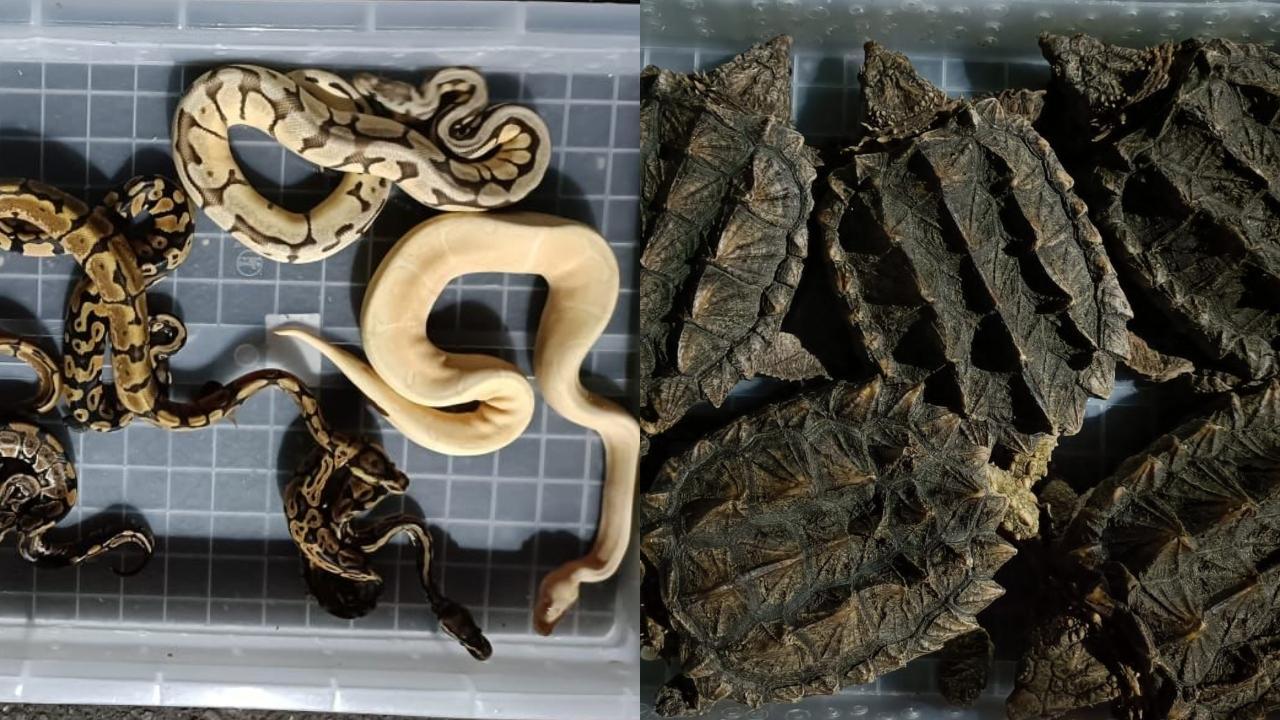The image depicts two distinct sections, each showcasing a different set of animals contained within bins with distinctive plaid-patterned tiles at the bottom. On the left side, there are about five diverse snakes, each exhibiting unique patterns and colors. Notably, there is a large, fully white snake and another white snake with brown stripes. Additionally, there are smaller snakes with intricate patterns, including one with brown spots and black dots, as well as a medium-sized brown snake with light black undertones and dark speckles. The edges of the bin have longer grey tiles, and the scene resembles a shower tray with very small, dark grey square tiles and light grey grouting. 

On the right side of the image, a similar bin houses what appear to be five unusual tortoises or snapping turtles. These turtles are dark brown, greenish, and grayish in color, with very scaly and spiky shells, featuring pointy heads. They are stacked on top of each other, making it difficult to discern individual features. The sides of this bin are made of perspex with small holes. While there is no textual information on the image, the setting suggests it might be a lab or an animal rescue facility.